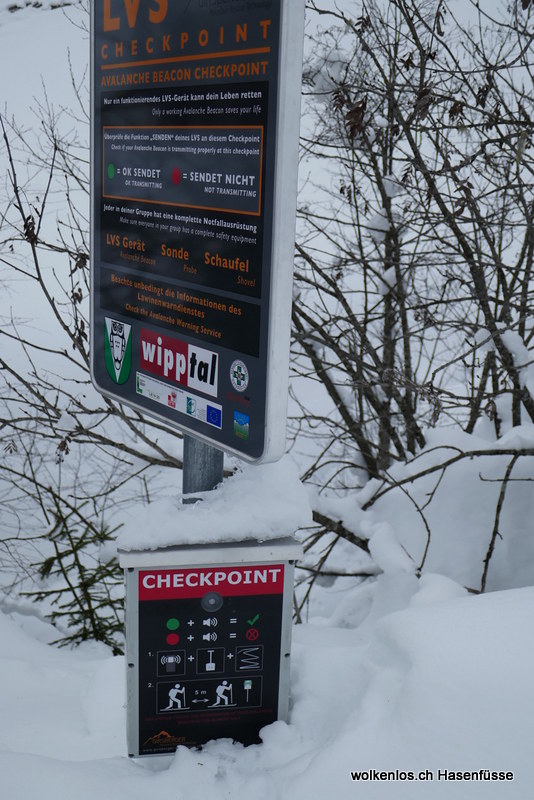In this outdoor winter scene, a thick blanket of snow covers the entire landscape, creating a stark white foreground littered with barren branches devoid of leaves, indicative of the cold season. Positioned amidst this snowy expanse are two rectangular signs—one large and mounted atop a metal pole, the other smaller and partially embedded in the snow. Both signs feature black centers bordered with white, overflowing with information in a foreign language, likely German, about an avalanche beacon checkpoint. The larger sign reads "LVS checkpoint" and "avalanche beacon checkpoint," with instructions and indicators such as "green - okay, transmitting" and "red - not transmitting," suggesting it’s an area for assessing avalanche beacons' functionality. The smaller sign below mirrors this theme, displaying "checkpoint" along with a red bar at the top, and features various icons, including a hiker wielding a stick. Snow partially obscures parts of the signs, emphasizing the heavy winter setting, and a faint watermark reading "wolkenlos.ch hasenfuseh" is visible on the bottom right of the smaller sign.